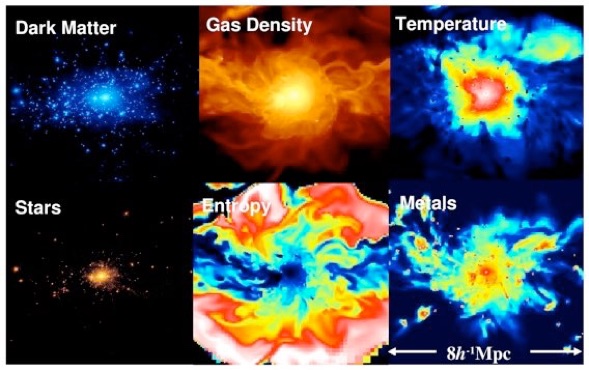This image is a composite of six scientific visualizations, each representing different cosmic properties:

1. The first photograph, titled "Dark Matter" in white font, depicts the vast expanse of space bathed in a subtle blue hue. Amidst this backdrop, a section illuminated in blue reveals a cluster of stars surrounded by glowing blue plasma.

2. The second photograph, labeled "Gas Density" at the top, vividly displays swirls of orange gaseous formations. At the heart of these swirling gases, a bright light radiates intensely.

3. The third photograph, marked "Temperature" at the top, features a cloud-like shape. The outer edges of this shape are cloaked in blue, transitioning to gradients of yellow, aqua, and orange towards the center, which culminates in a bright white core.

4. The fourth photograph, entitled "Stars," showcases a collection of orange stars scattered across the expanse of space. Dominating the center of this celestial assembly is a particularly bright orange star.

5. The fifth photograph, with the caption "Entropy," presents a mesmerizing array of swirling gas formations. This intricate display blends hues of red, yellow, aqua, and royal blue, creating a dynamic and colorful pattern.

6. The final photograph, titled "Metals" in white font, stands out against a dark space background. It features intricate shapes formed from gases in shades of royal blue, aqua, yellow, orange, and dark orange. At the bottom of this composition, the text "8H-1MPC" is presented in white, flanked by arrows extending outward from either side of the image.

Together, these images provide a detailed and colorful visualization of various cosmic phenomena, from dark matter and gas density to temperature, stars, entropy, and metallic elements in the universe.